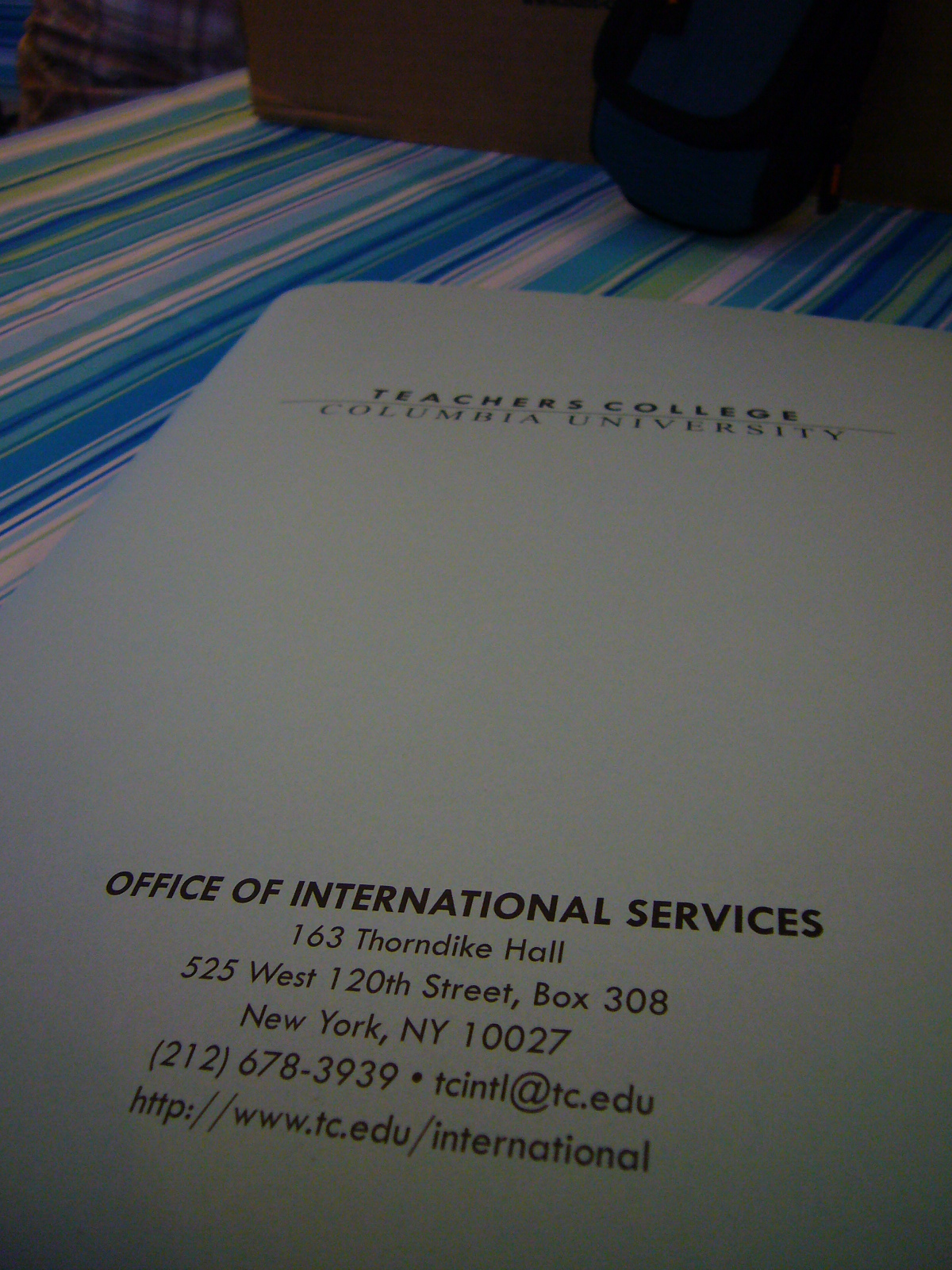The image depicts the front cover of a white brochure for Teachers College, Columbia University. The brochure, simply designed with black text, is lying on a vibrant, colorful striped tablecloth featuring white, blue, royal blue, light blue, and green stripes. The top section of the brochure prominently displays "Teachers College," followed by a thin line and "Columbia University." The bottom section provides detailed contact information: "Office of International Services, 163 Thorndike Hall, 525 West 120th Street, Box 308, New York, New York 10027," along with a phone number, "(212) 678-3939," an email address, "tcintl@tc.edu," and a website link, "http://www.tc.edu/international." Additional elements in the image, such as a data projector, a box, and a vinyl lunch box, are partially visible on the table.